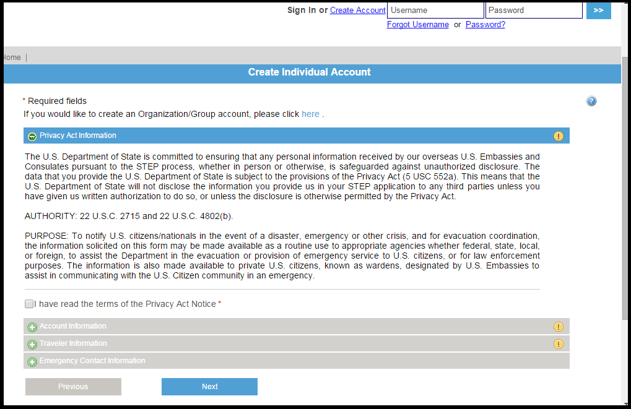The image depicts a website registration page set against a white background. At the top of the page, there's an option to "Sign In" in black text and "Create Account" in blue, which is hyperlinked. 

Below that, two input fields are labeled: the first says "Username" and the second says "Password." Adjacent to these fields is a blue button with two arrows pointing to the right. Just beneath the input fields, there’s a hyperlinked text in blue stating "Forgot Username or Password?"

Following this section, there's a gray banner labeled "Home," and below it, a blue banner that reads "Create Individual Account" in white print centered within it. 

Under this, a disclaimer in black text with an asterisk indicates that some fields are required. The text further explains that to create an organization or group account, one should click a hyperlinked "here" in blue print.

Towards the bottom, another blue banner states "Privacy Act Information," which briefly describes its purpose related to the US Department of State. Beside this, there is a checkbox labeled "I have read the terms of the Privacy Act notice."

Further down, sections titled "Account Information," "Traveler Information," and "Emergency Contact Information" are listed. Below these sections are two navigational buttons: "Previous" and "Next," with the "Next" button highlighted in blue.